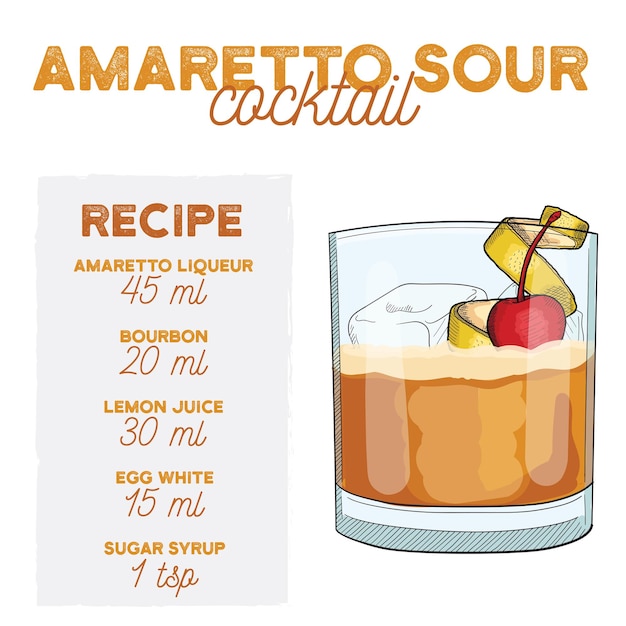This image presents a detailed recipe for crafting an Amaretto Sour Cocktail. At the top, the title "Amaretto Sour" is prominently displayed in large orange letters, with the word "Cocktail" below in cursive, darker orange text. The left side features a vertical gray box labeled "Recipe" in bold orange letters. Within this box, the ingredients and their respective amounts are listed in dark orange text: 

- Amaretto Liquor: 45ml
- Bourbon: 20ml
- Lemon Juice: 30ml
- Egg White: 15ml
- Sugar Syrup: 1 tsp

On the right side of the image, there is a cartoon-style drawing of a cocktail glass filled with a vibrant orange beverage. The glass is half-filled with a brown liquid and topped with a frothy, beige foam. Adorning the drink are two distinct garnishes: a red cherry positioned on the right side and a twist of yellow lemon peel to its left. Behind these garnishes and towards the back of the glass are two visible ice cubes. This depiction serves as a visual guide for creating the Amaretto Sour Cocktail.